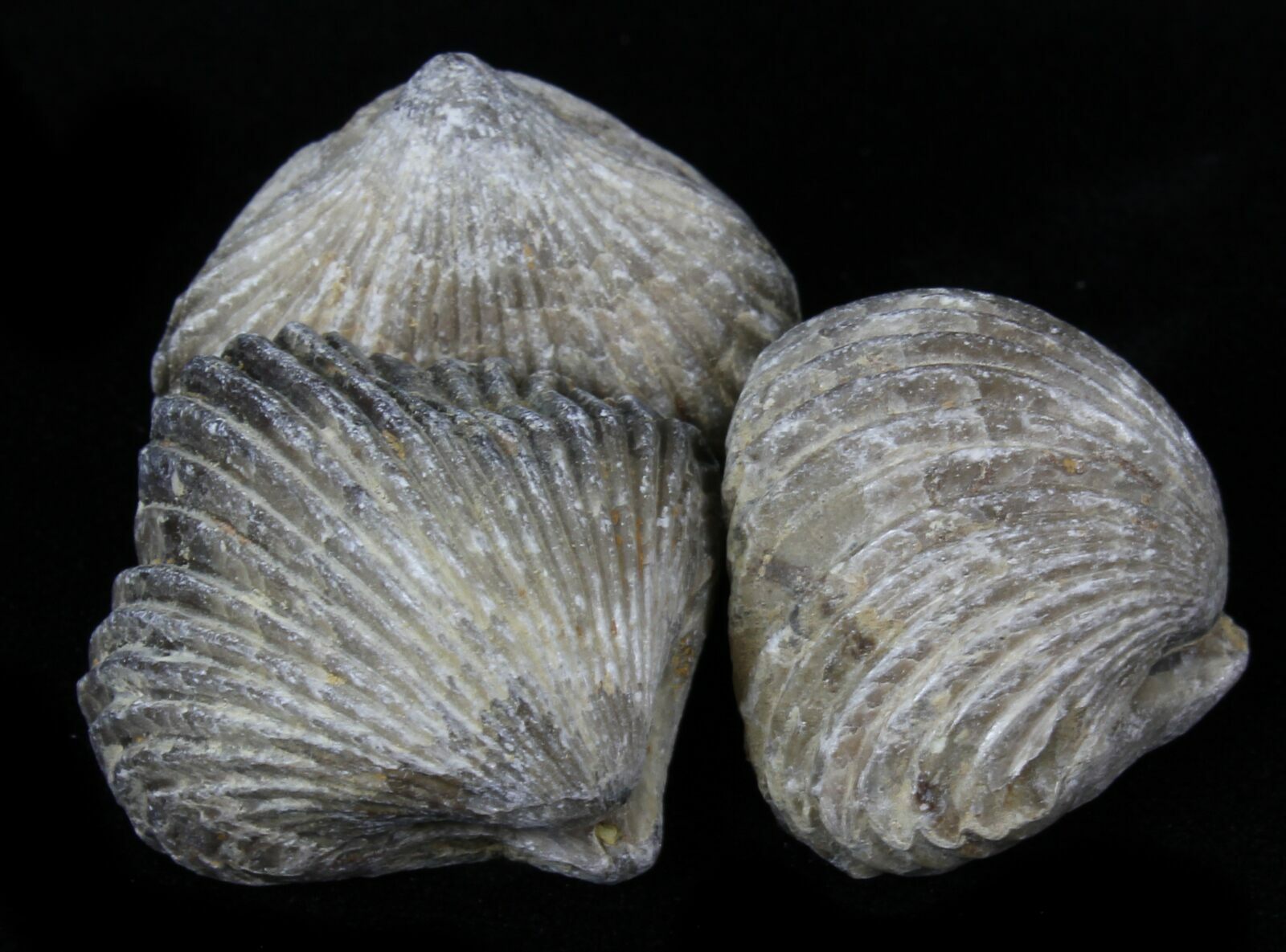The image showcases a photograph of three ancient-looking seashells displayed as an exhibit. The seashells are meticulously arranged on a completely black surface, which accentuates their features. Each shell varies slightly in color and texture; the one on the left in the front is predominantly gray with dark gray and black edging, while the two on the right have a tannish gray-brown hue. The leftmost shell points towards the upper left, the right shell points to the left, and the top shell on the left points downward. The shells appear dry and stony, giving them a petrified look, as though they might be stone sculptures. The ridges on the shells are visibly distinct, with the right shell featuring wider, more curved ridges compared to the closer-set ridges on the two left shells.